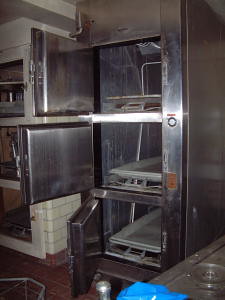This slightly dark and detailed color photograph appears to capture an industrial indoor setting which closely resembles a morgue. The primary focus is a large, stainless steel appliance dominating the right-hand side of the image, possibly used for refrigeration or storing bodies. This silver machine has three levels with doors wide open, revealing empty chambers each fitted with a sliding, light gray metal tray. A bright light source is reflecting off the machine, enhancing its metallic finish. To the left of the refrigerator unit, there is an adjacent white porcelain or stainless steel cabinet. The background wall is tiled in white with dark grout and is bordered by a reddish-brown trim similar to the tiled flooring.

In the foreground, occupying the bottom right-hand corner, there is a part of a metal table with a pair of blue plastic gloves resting on it. There also appears to be a small glass or clear container nearby. A hint of another blue object barely visible lies at the edge of the frame. The overall color palette of the image features dominant shades of silver, grey, white, and dark brown, illuminating the sterile and clinical atmosphere of the space.